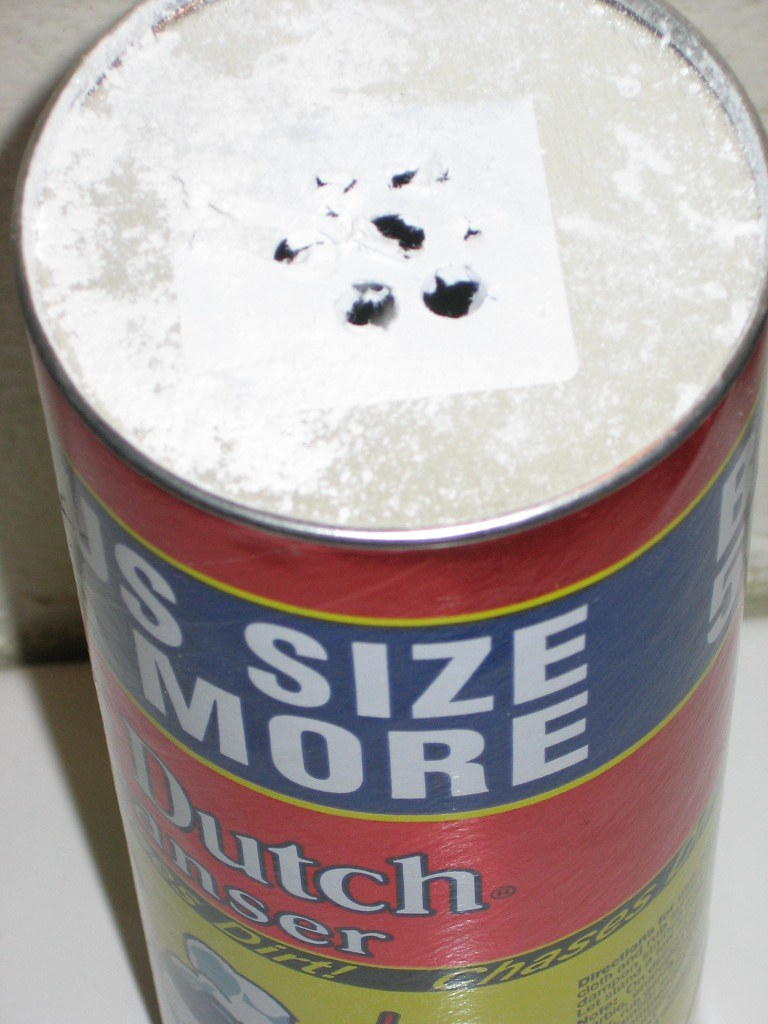This image is a close-up view of a vintage metal can of powdered cleaner. The label on the can prominently features the partially visible word "cleanser," specifically displaying the letters "N-S-E-R." Above the text, it reads "Dutch," potentially indicating the brand or origin. The can promises to "chase dirt away." The image is taken from an angle above the can, showing a white seal on the top that has been punctured with a series of holes, allowing the powdery substance to be dispensed. The label itself is visually striking, adorned with an array of colorful stripes in red, yellow, blue, black, and yellow, each stripe featuring different text or design elements in varying typefaces. Notably, the words "size," "more," "Dutch," "cleaner," and "dirt" differ in both font and size, adding a dynamic, eye-catching quality to the overall design.